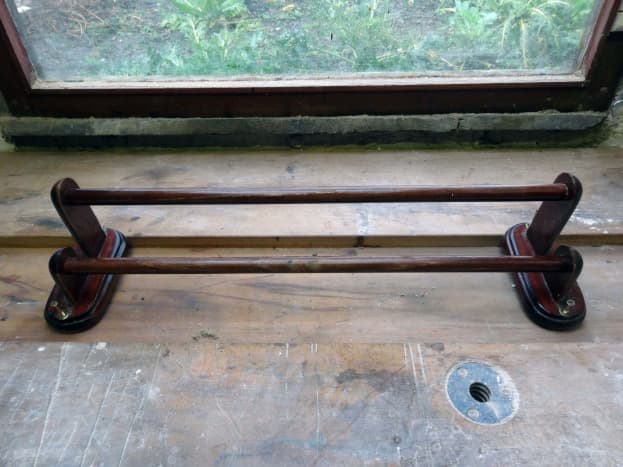This image displays an oddly angled scene, making it challenging to discern the exact perspective or purpose of the objects depicted. On the top, there's a section of a window framed in brown, which seems to open outwards. Through the window, you can glimpse green leaves and natural scenery, although it's difficult to identify specific outdoor details. Below the window, a structure resembling a hanger or rack is mounted. The base appears to be pill-shaped and is secured to what looks like a gray cement surface. This rack consists of finished, dark brown wooden poles, with one rod positioned higher than the other. 

The polished wooden material suggests it might be a tie rack or towel hanger, though its unusual placement adds to the ambiguity. Interestingly, the presence of a silver circle, perhaps a screw or metal fixture, is also noted on the cement surface beneath the rack. The overall impression is of a well-crafted wooden hanger structure set against a mix of wooden and stone elements, contributing to the photograph's mysterious and perplexing nature.